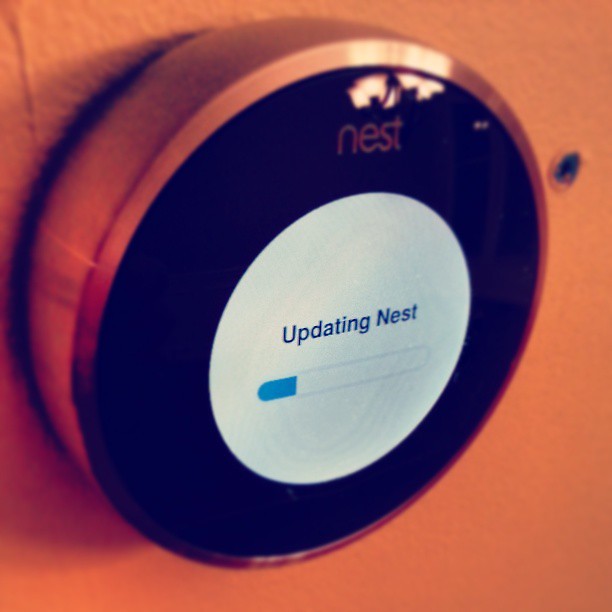This close-up photograph captures a Nest thermostat from a slightly elevated, left diagonal angle, emphasizing its prominent presence in the frame. The backdrop features a vibrant orange wall, which contrasts with the thermostat's sophisticated design. The device itself boasts a bronze rim encircling a sleek black display. At the top center of the display, "nest" is elegantly written in white. The screen is actively updating, indicated by a central white circle and the text "Updating Nest" in black, situated above a blue progress bar approximately 10% complete. Notably, to the right of the thermostat, there’s a visible hole in the wall, possibly from a previous doorbell or thermostat installation, adding a touch of reality to the scene.